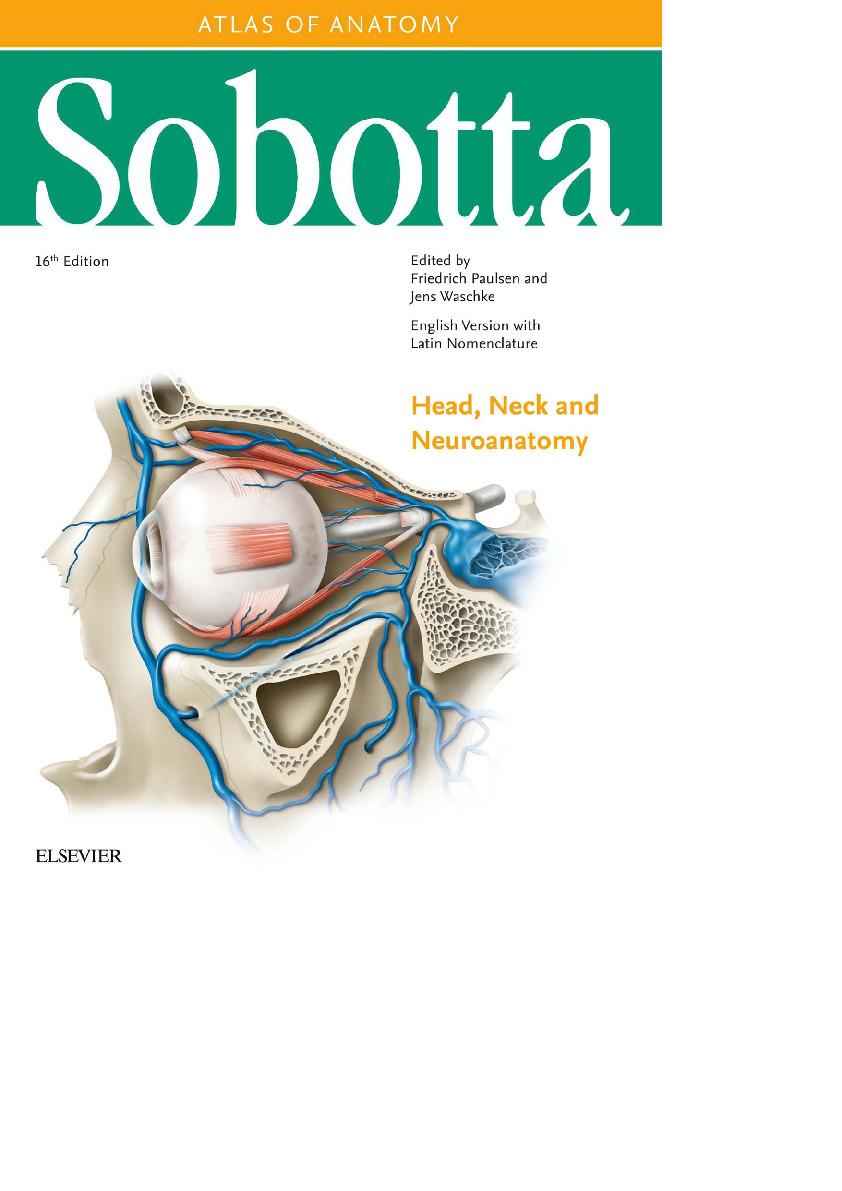This is the cover page of the 16th edition of the textbook titled "Atlas of Anatomy, Sobotta," edited by Friedrich Paulsen and Jens Waschke. The cover features a minimalist design on a plain white background. It has two headers at the top: the first is an orange banner with small white print reading "Atlas of Anatomy," positioned about a quarter of an inch down from the top, followed by a thin horizontal white line. Below this is a green banner, approximately three-quarters of an inch in height, with bold white text that reads "Sobotta," extending across the width of the cover. The letters in "Sobotta" touch the bottom of the green banner, blending into the white background below. Towards the upper left corner of the cover, there is black print stating "16th Edition," and towards the right, it mentions "Edited by Friedrich Paulsen and Jens Waschke." Beneath, it indicates "English version with Latin nomenclature" and in orange print, it specifies "Head, Neck, and Neuroanatomy." The central illustration depicts a cross-section of a human eye facing left, revealing the internal skull area complete with blue veins and red nerves. In the lower left corner, the publisher "Elsevier" is mentioned in black print.